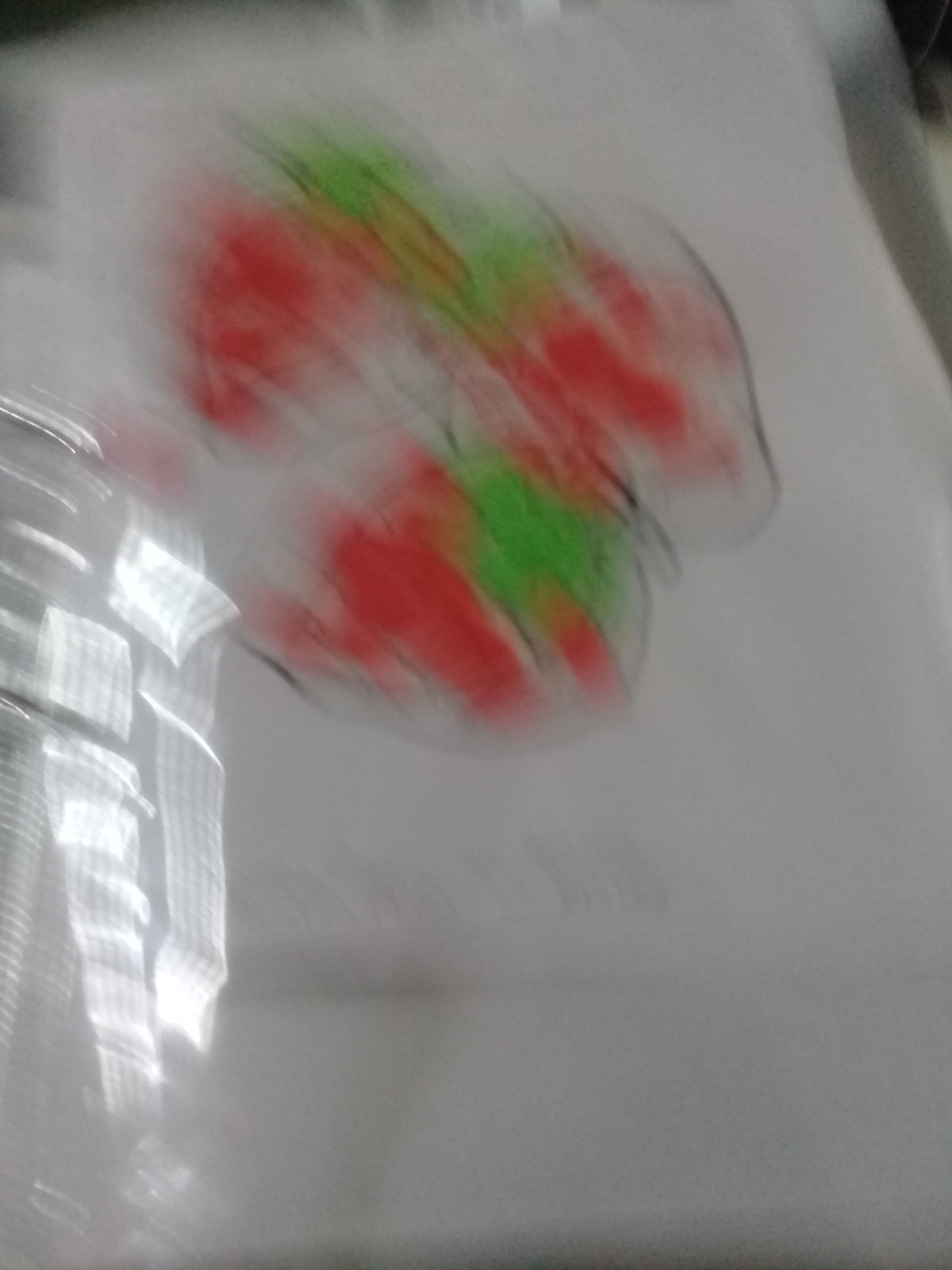A stark white concrete wall stands as a canvas for a charming artistic depiction, with a nearby window casting gentle light and forming gridded patterns of window panes across the surface. The artwork features large strawberries, each outlined in bold black lines and whimsically colored with streaks of red. The strawberries' green leaves and stems, similarly outlined in black, add to the playful yet imperfect aesthetic, with hints of green shading providing depth and character to the overall composition.